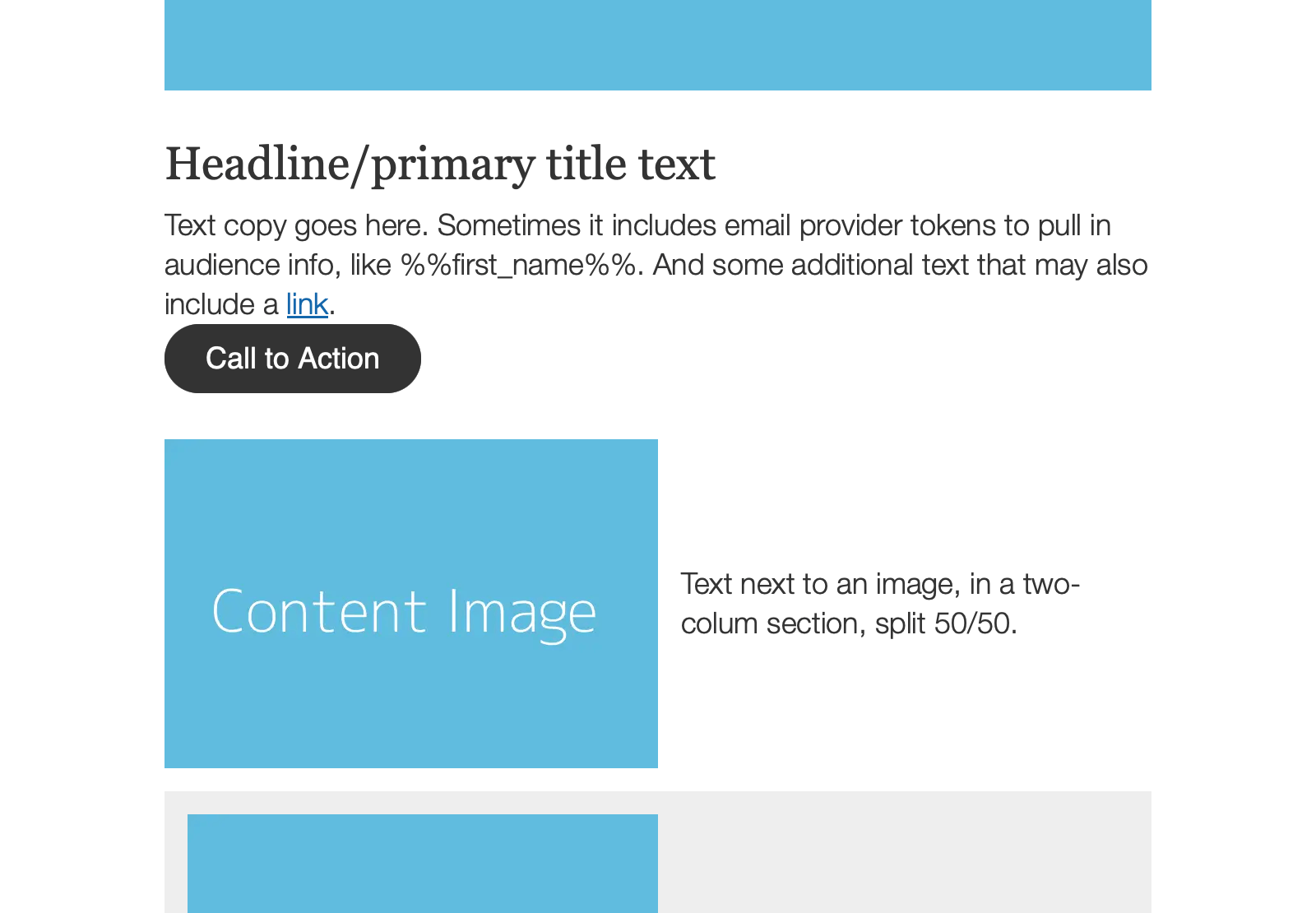This image is a screenshot of a software interface. At the very top of the screen, there is a medium, sky-blue bar stretching across the entire width, which is blank. Below this bar, the background shifts to white, where black text prominently reads "Headline/Primary Title Text." In smaller black letters, it says "Text copy goes here." Occasionally, placeholders like "%%FIRST_NAME%%" are used to personalize the content with audience information. This section may also include additional text and a hyperlink, with the link itself highlighted in blue to indicate its clickable nature.

Further down, there is a black oval button featuring the text "Call to Action" in white. Below this button, a horizontal sky-blue rectangle contains the text "Content Image" in white letters. Adjacent to this blue rectangle, on the white background, black text reads "Text next to an image in a two-column section split 50/50."

At the lower portion of the image, a gray bar spans across the screen. On the left side of this gray bar, there is another blue rectangle.